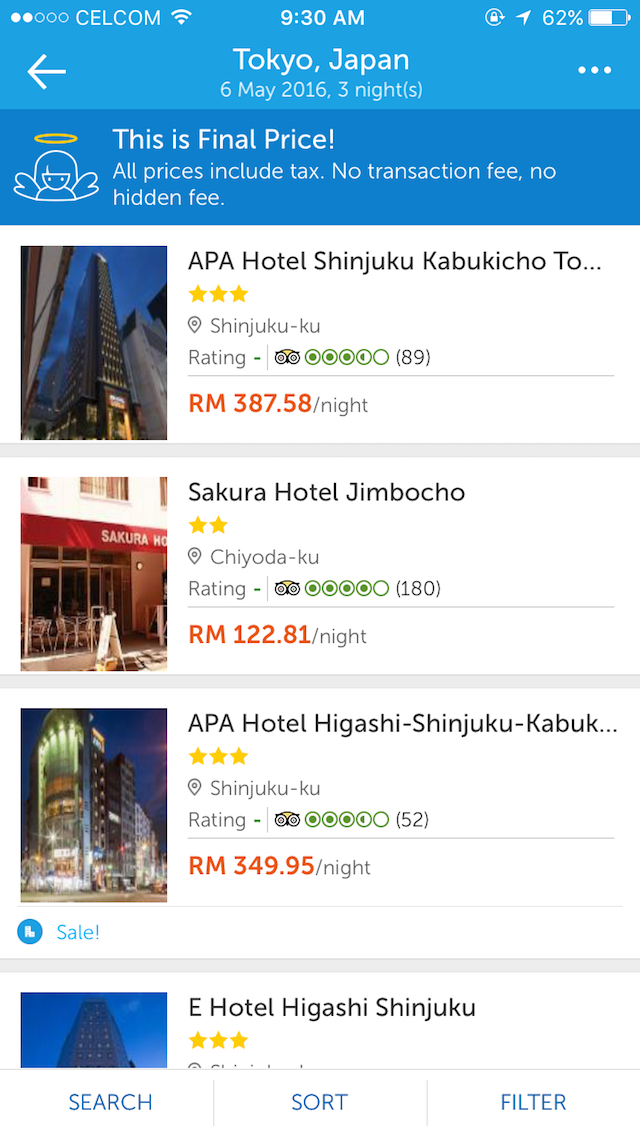In this image, you see a mobile phone screen displaying a booking interface for hotels. 

At the top left corner, the screen shows the cellular network labeled "Cell Comm" and a Wi-Fi signal icon. The time displayed in the middle is 9:30 a.m. On the top right corner, there is a battery life indicator showing 62% remaining.

Below this top bar, the screen reads: 
   
   **Location and Date Information:** 
   "Tokyo, Japan - 6 May 2016 for 3 nights." 

On the left side of this section, there is a left-pointing arrow, and on the right side, there are three vertical dots, typically indicating additional options or a menu. This section is set against a light blue background.

Below the location and date information, against a regular blue background, the following message is displayed:
   
   **Pricing Information:** 
   "This is the final price. All prices include tax, no transaction fee, no hidden fee." 
   
To the left of this text, there is a logo resembling a halo.

Further down, the names and details of four hotels are listed:

1. **APA Hotel Shinjuku-Kabukicho:**
   - Rating: 3 stars.
   - Price: Displayed in red beneath the hotel name.
   - An image of the hotel is to the left of the name.

2. **Sakura Hotel Jimbocho:**
   - Rating: 2 stars.
   - Price: Displayed below the hotel name.
   - An image of the hotel is to the left of the name.

3. **APA Hotel Higashi-Shinjuku-Kabukicho:**
   - Rating: 3 stars.
   - Price: Displayed below the hotel name.
   - An image of the hotel is to the left of the name.

4. **E Hotel Higashi Shinjuku:**
   - Rating: 3 stars.
   - Price: Displayed below the hotel name.
   - An image of the hotel is to the left of the name.

At the bottom of the screen, there are options for searching, sorting, and filtering the hotel listings.